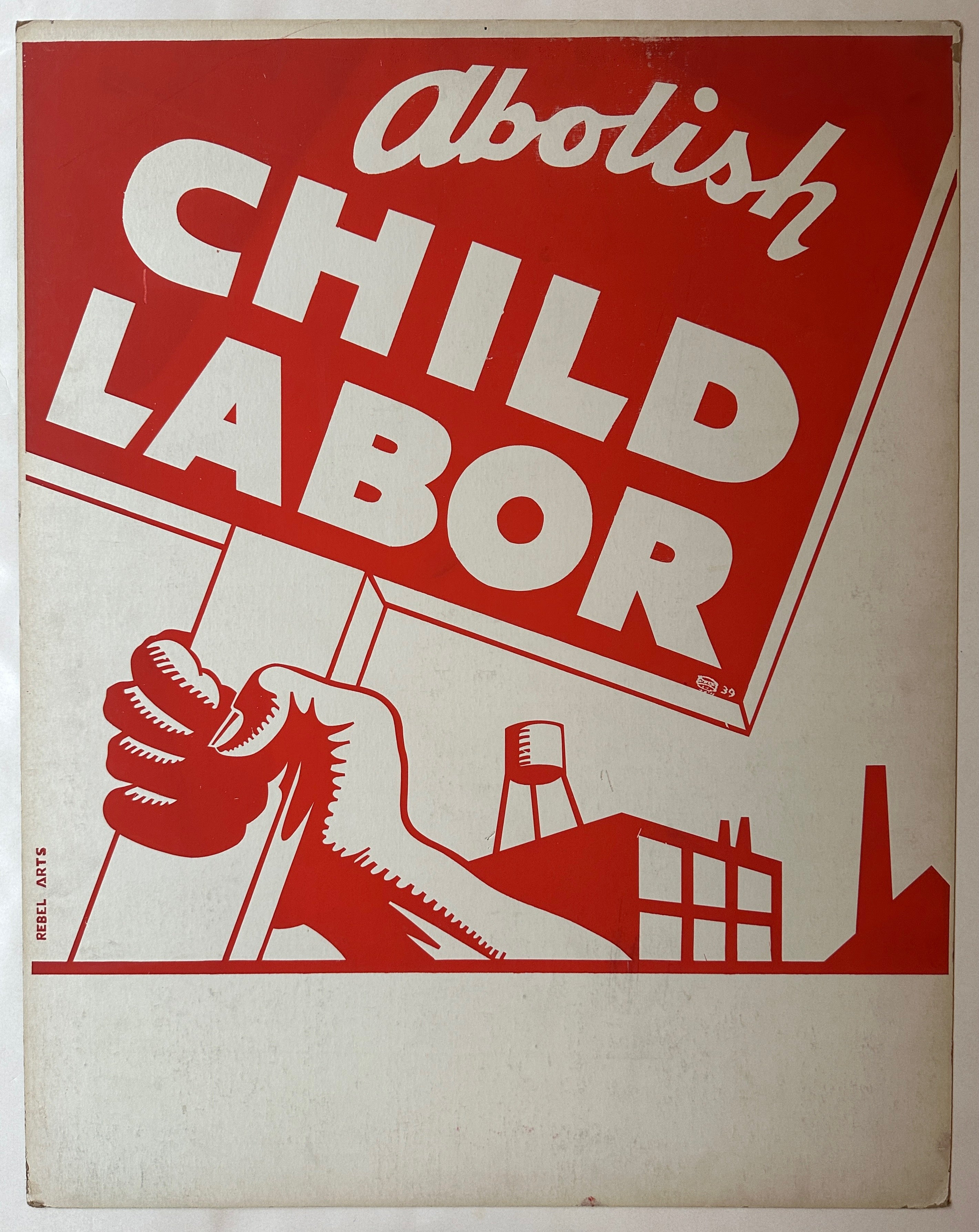This photograph captures a weathered, vintage political poster that appears screen-printed on white paper, showcasing wear typical of genuine use. The poster features a monochromatic red and white color scheme with bold, cartoonish details, reminiscent of woodcut block or Art Deco styles. Dominating the image is a stylized hand gripping a wooden picket sign, emblazoned with the slogan: "Abolish Child Labor." The word "Abolish" is elegantly cursive, while "Child Labor" is in commanding block letters. The background depicts graphic images of a simplistic warehouse or factory, complete with a tall smokestack and a water tower. Additional fine print running vertically near the hand reads "Rebel Arts," likely referencing the creator. Small text in the bottom right corner displays the number 39, adding a touch of specificity to this evocative representation of labor activism.